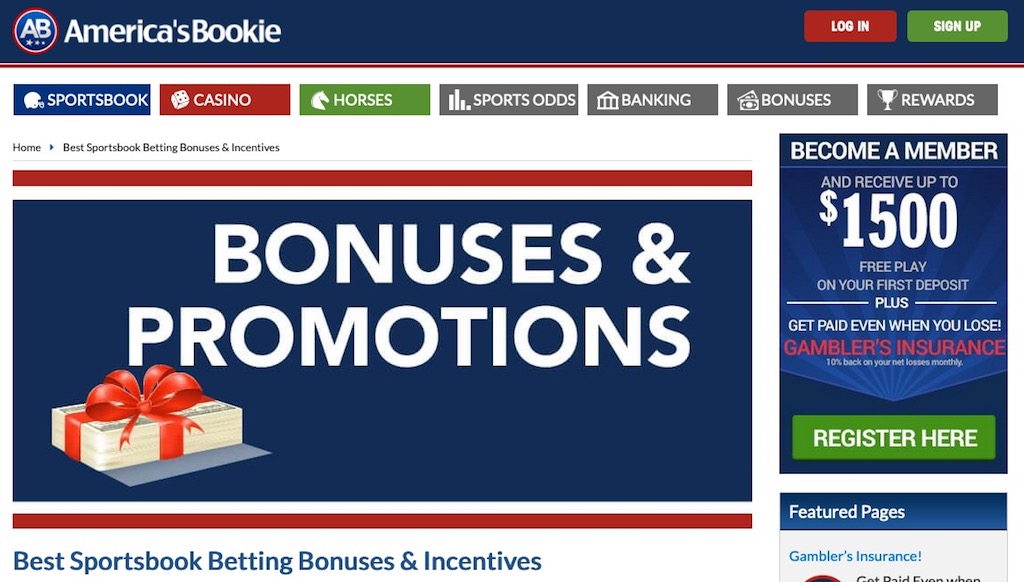The top-left corner of the image features a logo labeled "AB," alongside a star that reads "America's Bookie." On the right, there are red and green buttons labeled "Login," with the text "Login" displayed within a green square. Along the top left, the options are color-coded: "Sportsbook" in blue, "Casino" in red, and "Horses" in green.

Beneath these options are four gray squares that lead to different sections: "Sports Odds," "Banking," "Bonuses," and "Rewards." Additionally, navigation options are listed including "Home," "Best Sportsbook," "Betting," "Bonuses," and "Incentives," along with a prominent red rectangle.

The central portion of the image showcases a large banner titled "Bonuses and Promotions," featuring a stack of cash tied with a red ribbon. Below this image, the text highlights "Best Sportsbook, Betting, Bonuses, and Incentives."

On the top right, there's a call-to-action box that entices viewers to become members, offering up to $1,500 free to play on their first deposit. It also mentions "Gambler's Insurance," which provides 10% back on internet losses monthly. This section prompts users to "Register here."

Below this, the text "Featured Pages" includes "Gambler's Insurance," explaining that users can "get paid even when" against a backdrop of notable site features like "Sportsbook, Casino, Horses, Sports Odds, Banking, Bonuses, and Rewards." The emphasis throughout the image is on "Bonuses and Promotions," highlighting the various incentives the site offers.

Overall, the image serves as an advertisement for a sports betting site, detailing sections like "Sportsbook, Casino, Horses, Sports Odds, Banking, Bonuses, and Rewards" and prominently featuring their promotional offers.